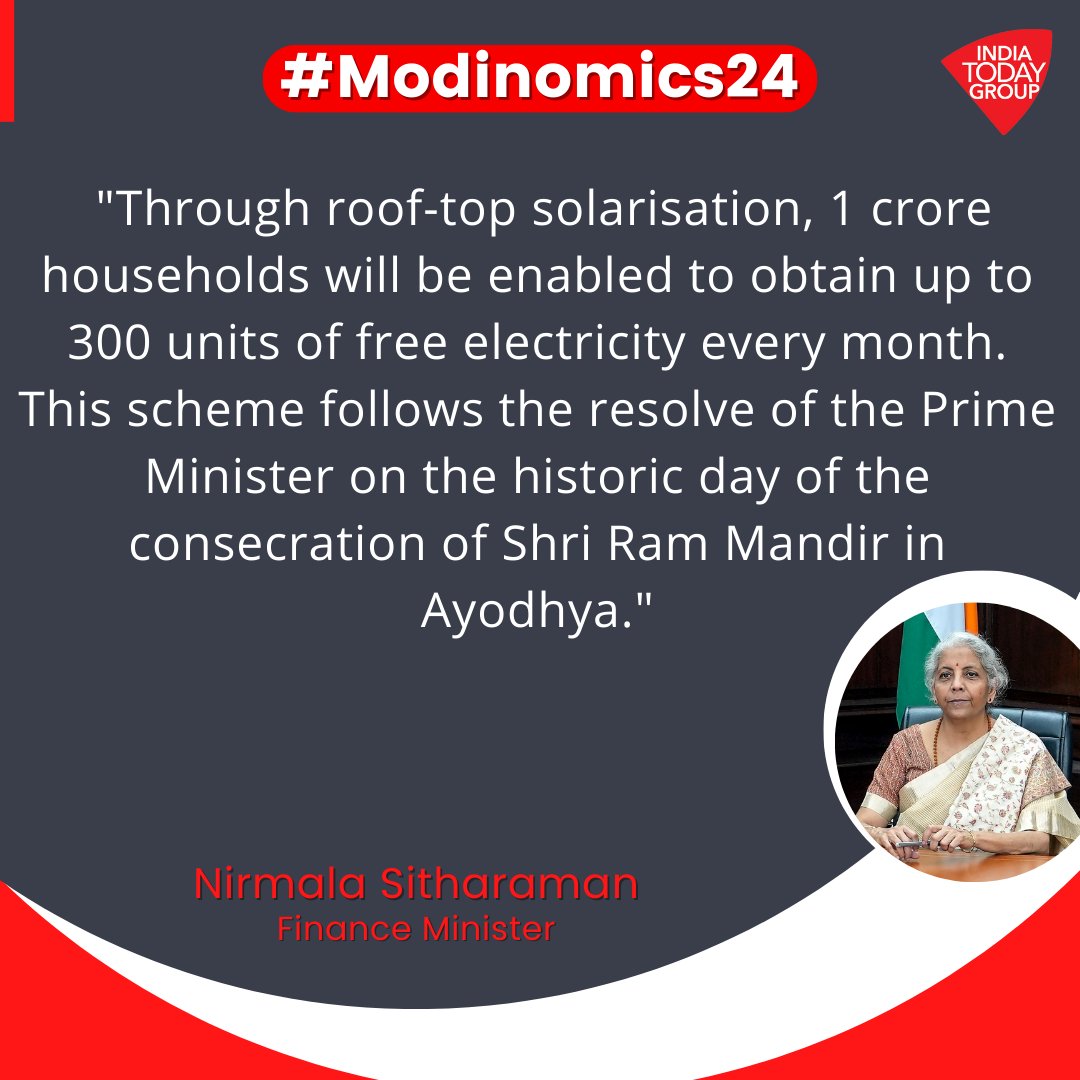The image appears to be a print ad or a web page advertisement by the India Today Group, featuring a photograph of Nirmala Sitharaman, the Finance Minister of India. The background is predominantly a basic black or gray color with accents of red and white text. In the upper right-hand corner, the India Today Group logo is displayed. A notable element at the top is the hashtag "Modinomics 24," referring to policies associated with Prime Minister Modi.

Central to the ad is a quote from Nirmala Sitharaman: "Through rooftop solarization, one crore households will be enabled to obtain up to 300 units of free electricity every month. This scheme follows the resolve of the Prime Minister on the historic day of the consecration of Shri Ram Mandir in Ayodhya." The text, in striking white and red, emphasizes the government's initiative to promote solar power in India.

At the bottom quarter of the picture, there are decorative swishes in white and red, adding a visual element to the otherwise text-focused advertisement. The depicted Indian woman in the bottom right corner, likely Nirmala Sitharaman, is wearing a brown outfit, lending a personal touch to the advertisement.